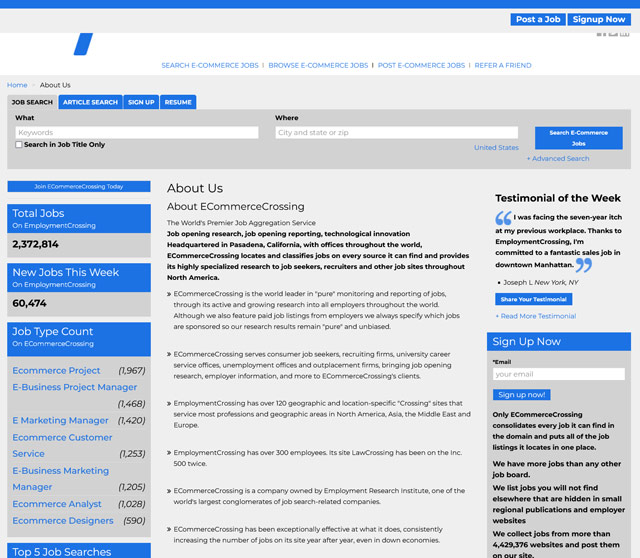This image showcases a navigational interface for an e-commerce job search website. The top section prominently features menu options: "Search E-commerce Jobs," "Browse E-commerce Jobs," "Post E-commerce Jobs," and "Refer a Friend." Additionally, the top-right corner includes quick access buttons for "Post a Job," "Sign Up Now," "Home," "About Us," "Job Search," "Article Search," "Sign Up," and "Resume."

Below the navigation bar, search fields for job hunting are visible, allowing users to enter "What" (keywords) and "Where" (city and state or zip code). There's an option to narrow the search to "Job Title Only."

The main body of the image promotes joining the website with a call to action: "Join E-commerce Crossing Today." Statistics are highlighted, noting "Total Jobs on Employment Crossing: 2,372,814" and "New Jobs This Week on Employment Crossing: 60,474."

Further detailed is a section displaying job type counts on E-commerce Crossing and featuring a "Testimonies of the Week" spotlight. A user testimonial reads: "I was facing the 7-year age gap at my previous workplace. Thanks to Employment Crossing, I'm now committed to a fantastic sales job in downtown Manhattan." The testimonial is attributed to Joseph L. from New York.